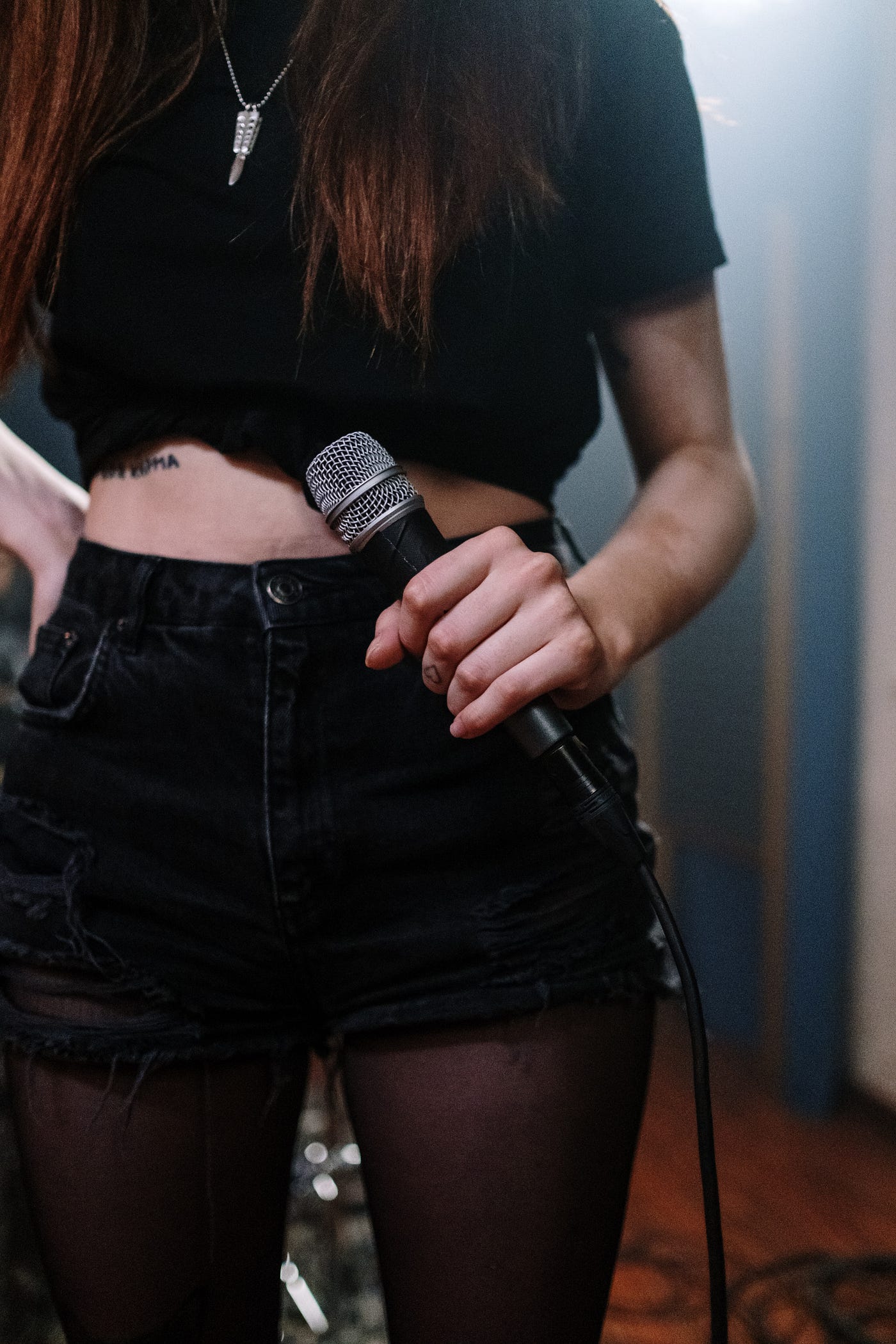In this color photograph, which is portrayed in a portrait orientation with a focus on realism, a singer stands on a dimly lit stage with a single bright light source positioned above her on the left. The image captures her from the top of her shoulders down to about her knees, with her standing slightly cropped off on the left side. She has long, straight, brownish-reddish hair flowing down to midway of her torso and wears a silver necklace around her neck. The singer is dressed in a very short, black, cropped shirt that reveals part of her stomach above her belly button, black ripped denim shorts that rise above her belly button, and black stockings underneath. Her left hand holds a microphone near her waist, its cord wrapped around her hand, while her right hand rests on her hip, revealing a small black tattoo on her right stomach area, which includes the word "Yuma." The background features a reddish-brown carpeted floor and a blue and white striped wall.